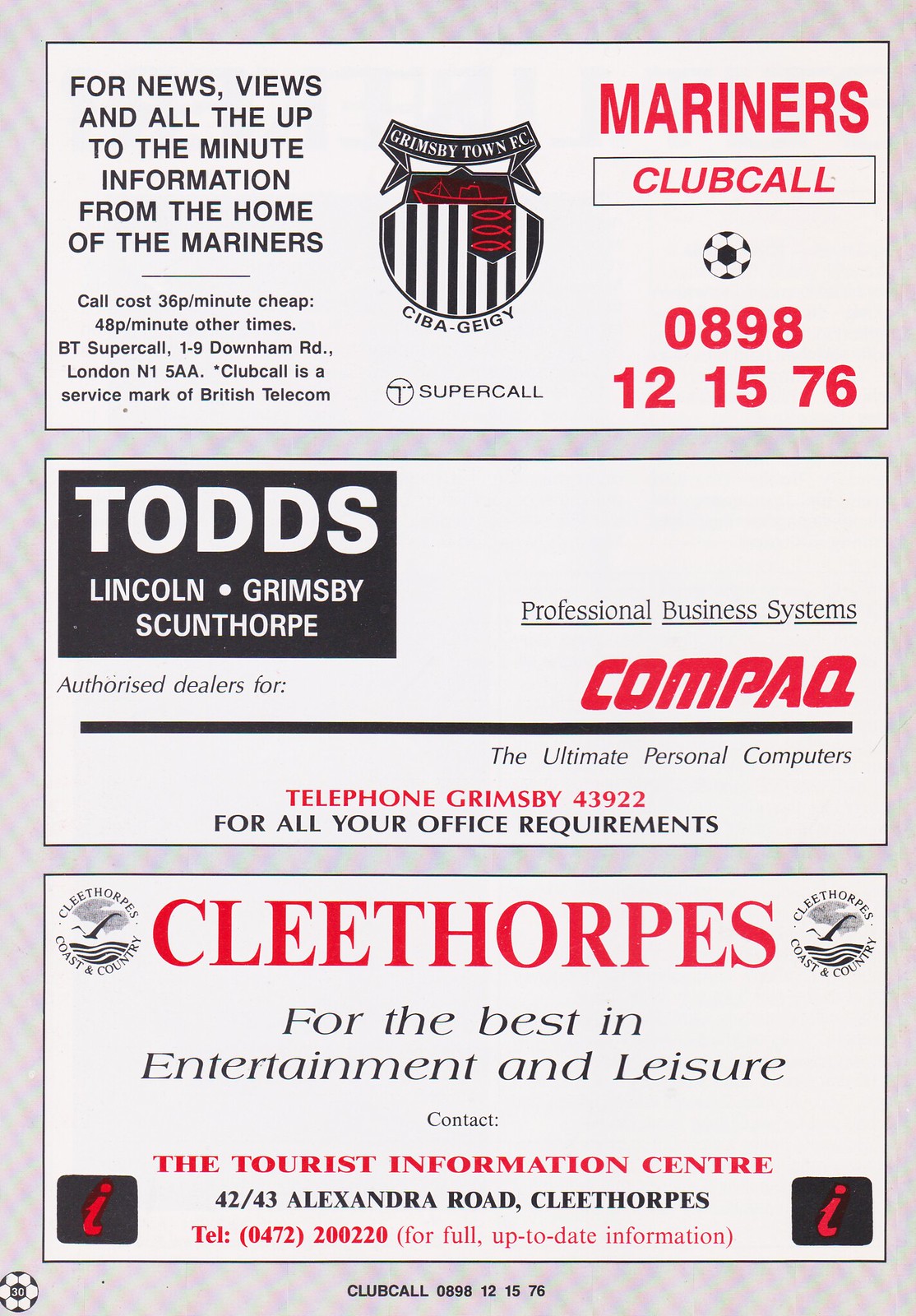The image is a page from an old magazine, featuring three distinct advertisements against a blue-gray background. Each ad is sectioned off in its own bordered box. The top advertisement, outlined in black with a white background, is for the Mariners Club. It prominently displays "Mariners Club Call 0898-1215-76" in red, beside a logo. The ad promises "news, views, and all the up-to-the-minute information from the home of the Mariners" and includes a note about call costs. Below this, the second advertisement is for Todd's professional business systems, specializing in Compaq computers. It reads "Todd's Lincoln Grimsby Scunthorpe" and highlights "Authorized Dealer for Compaq, the ultimate personal computers" in red, followed by the phone number "Grimsby 43922" for office requirements. The final box, with "Cleethorpes" in bold red text flanked by two logos, promotes local entertainment and leisure. It invites readers to "contact the Tourist Information Centre, 42-43 Alexandra Road, Cleethorpes" with the telephone number "0472-200-220" for more information.